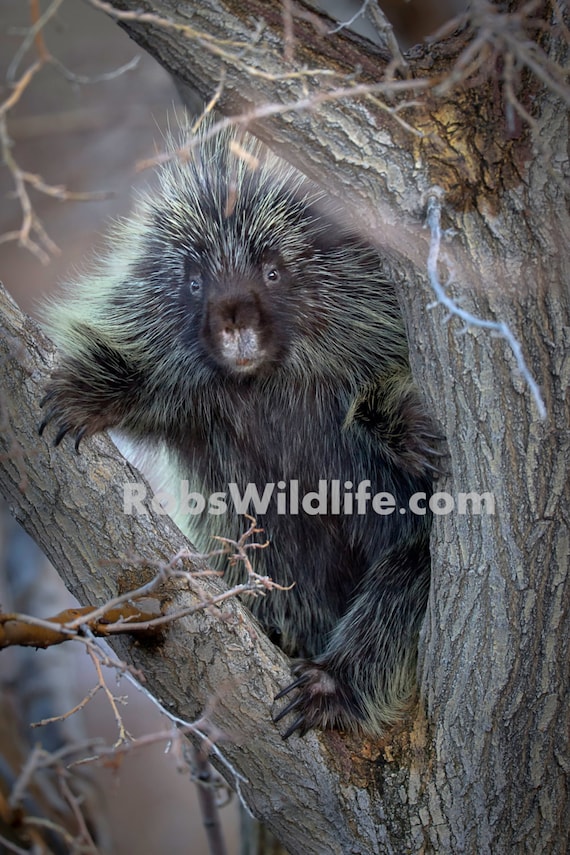The daytime image takes place in a forest setting, dominated by a bare tree situated prominently on the right-hand side. This tree, devoid of leaves, features a dense network of branches and twigs. In the tree, there's an endearing animal, a hedgehog, gripping the Y-shaped junction of two branches with its front legs splayed on either side. The hedgehog, characterized by its blackish-brown fur and light greenish-yellow tinted quills, displays a distinctive white patch around its nose and mouth. Its fur is very shaggy and bushy, and it also has notably long claws. The branches have thick, furrowed light-gray bark, with some parts appearing brown. The hedgehog appears to gaze directly towards the viewer, amidst the surrounding intricate web of twigs and branches displayed prominently at the top and bottom left of the image. Overlaid near the hedgehog's tummy area are the words "robswildlife.com" in light gray letters.